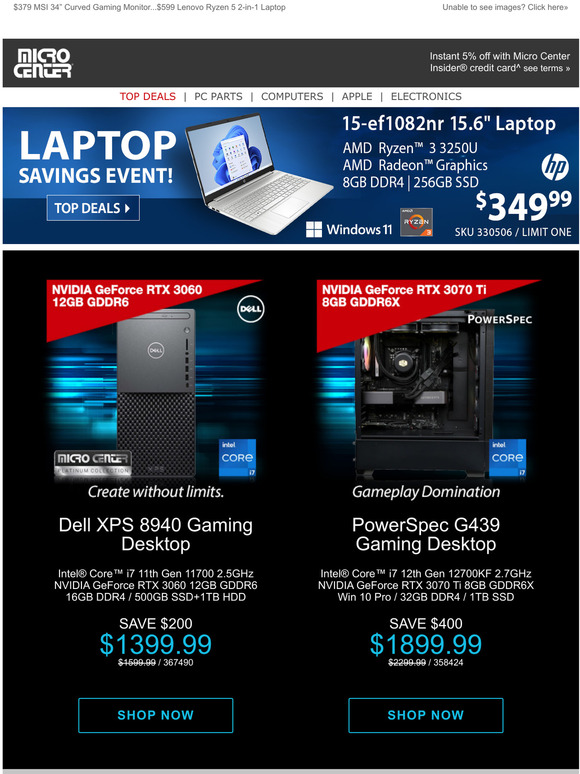The image showcases a web page from the Micro Center store, primarily featuring various tech deals against a mostly black backdrop with minimal white sections. At the top left, the screen reads "$379 MSI 34-inch Curved Gaming Monitor ... $599 Lenovo Ryzen 5 2-in-1 Laptop." On the upper right, there's a prompt: "Unable to see images? Click here." Below this, the "Micro Center" logo appears in white on the upper left, and on the upper right, you find the message "Instant 5% Off with Micro Center Insider Credit Card. See Terms."

The web page is currently displaying the "Top Deals" section, highlighted in red. Additional categories such as "PC Parts," "Computers," "Apple," and "Electronics" are listed nearby. A blue banner with white text announces the "Laptop Savings Event."

An image of an open gray laptop, featuring a screen with a swirling blue design, showcases the following specs: "HP 15-EF1082NR 15.6-inch Laptop, AMD Ryzen 3 3250U, AMD Radeon Graphics, 8GB DDR4, 265GB SSD, Windows 11, $349.99, SKU 330506, Limit 1."

The page also features a gray Dell computer tower, adorned with the Dell logo and the Intel Core i7 badge, under the "Micro Center Platinum Collection." This product is described as a "Dell XPS 8940 Gaming Desktop:
- Intel Core i7 11th Gen 11700 2.5GHz
- NVIDIA GeForce RTX 3060, 12GB GDDR6
- 16GB DDR4, 500GB SSD + 1TB HDD
- Save $200.00."

The adjusted price of $1,399.99, from an original $1,500.00, is shown in blue.

Adjacent is another image featuring a PowerSpec G439 Gaming Desktop:
- Intel Core i7 12th Generation 12700KF 2.7GHz
- NVIDIA GeForce RTX 3070 Ti, 8GB GDDR6X
- Windows 10 Pro, 32GB DDR4, 1TB SSD
- Save $400.00."

This item is priced at $1,899.99, reduced from $2,200.00.

The promotional text and pricing details emphasize the major discounts available on laptops and gaming desktops, making it evident that this is an advertisement for a tech sale at Micro Center.